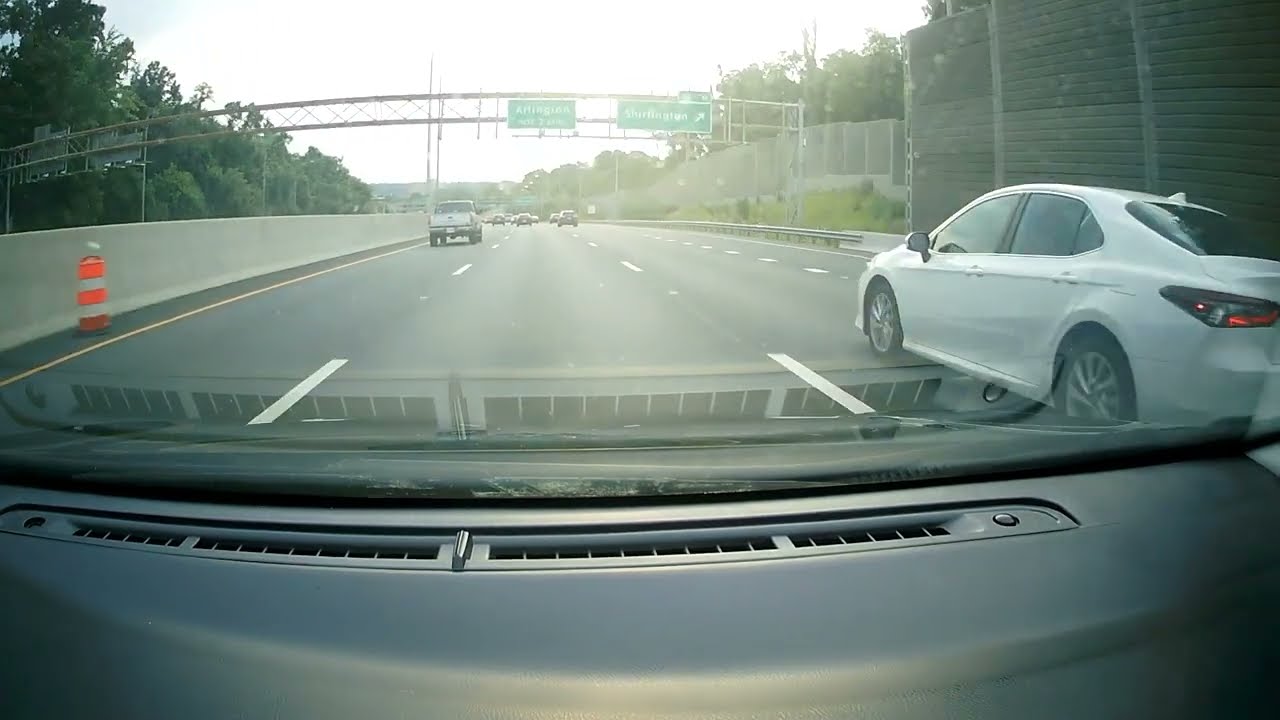This image depicts the view from inside a car looking out through the windshield onto a multi-lane highway. The dashboard, including the defroster grate, is visible at the bottom of the image. The car is traveling in the second lane from the left on a four-lane highway. To the immediate right of this car is a white sedan, visible from its bumper to its front. In front of the car and slightly to the left is the back of a pickup truck. Farther left, along the concrete barrier that runs parallel to the road, there is an orange and white striped construction barrel. 

Above the highway, there is a metal archway with green signs that have white lettering. The leftmost sign reads "Arlington, next 3 miles," with an exit indicator. The right side of the image shows more grass bordering the road, followed by a green barrier and a line of trees beyond. The background of the highway is filled with additional cars, though traffic appears to be moderate. The sky above is light blue, contributing to the overall palette of black, gray, white, orange, green, and light blue visible in the image.